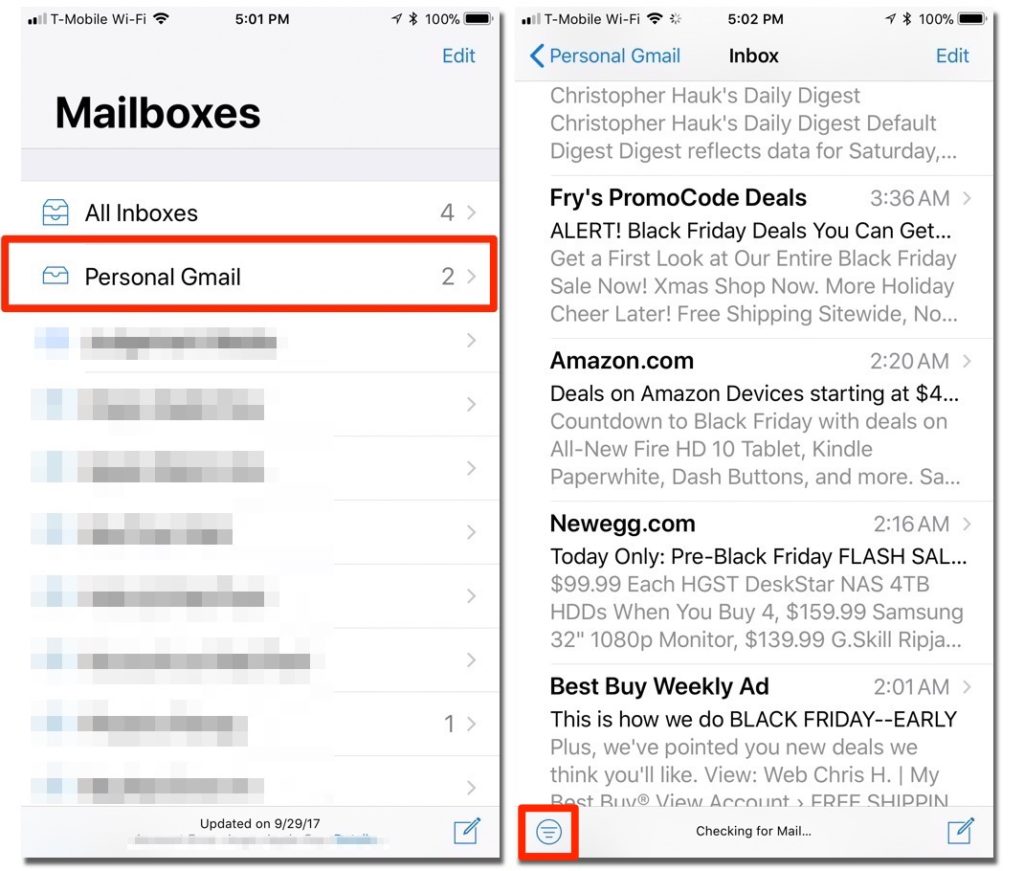The image consists of two side-by-side screenshots, each displaying different views of an email client. 

In the first screenshot, the left pane of the email client is visible. It features a section labeled "All Mailboxes" with a count of four. Below this, a "Personal Gmail" folder is indicated with a count of two emails. There are eight additional rows beneath "Personal Gmail," but these rows are blurred out and their details are not visible.

The second screenshot depicts the content of the "Personal Gmail" folder after being clicked. At the top, "Personal Gmail" and "Edit" are written in blue, highlighting that this folder is currently being viewed. Below this header, five emails are listed. The email subjects and timestamps are:
1. At 3:36 PM, an email titled "Fry's Promo Code Deal Alert."
2. An email from Amazon.
3. An email from Negwood.com labeled "Today Only."
These emails are all categorized as promotions. 

Additionally, there is a circle with three horizontal bars, which is surrounded by a red box to draw attention to this element on the interface.